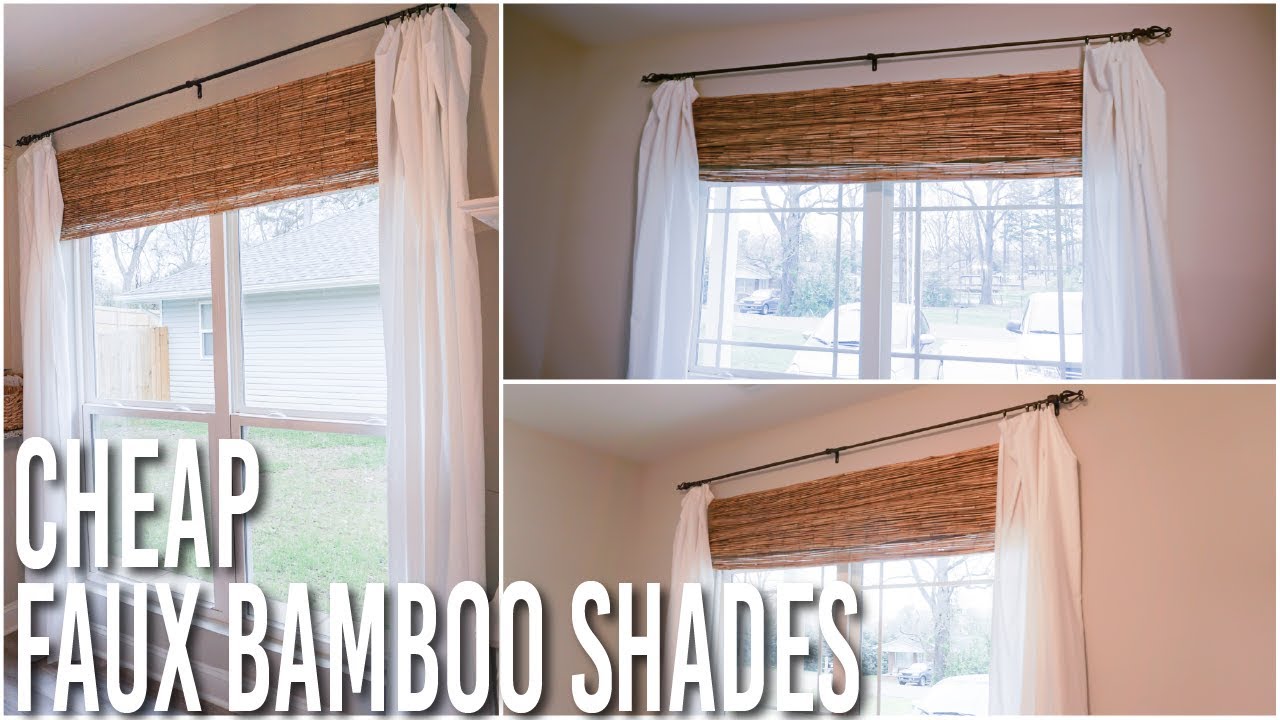The collage consists of three vertically rectangular photographs arranged with one larger image on the left and two smaller images stacked on the right. Each photograph depicts the same indoor scene featuring a window framed by light brown wood. The window is adorned with white curtains held by a skinny black metal rod, and a pulled-up bamboo shade at the top. The curtains are pushed to the sides, and through the window, one can see a yard with green grass and another house. 

The left image provides an angled view from the right side of the window, exposing a wide perspective of the scene outside. The top right image shows the top portion of the window from a frontal view, while the bottom right image emphasizes the top part from another right-side angle. The wall surrounding the window is painted a light peach-pink color with a white ceiling. The collage is framed with a thin white border, and at the bottom right corner, bold, all-capital white text with a drop shadow reads "CHEAP FAUX BAMBOO SHADES."